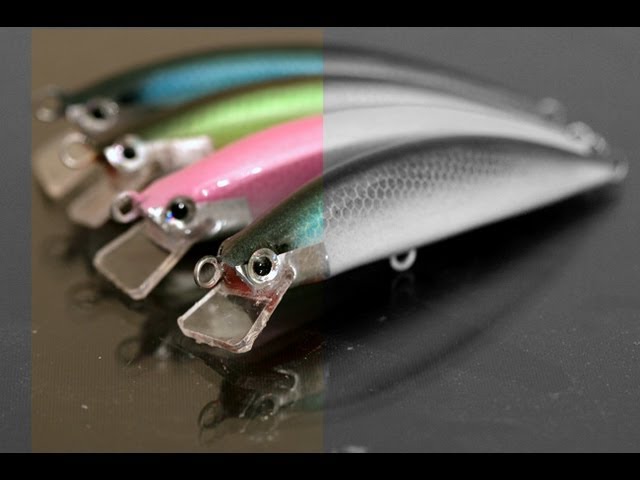The image is a close-up photograph of four artificial fishing lures, each distinctly colored and meticulously aligned on a shiny black surface that reflects their forms. The picture is uniquely edited with a clear dividing line; the left half displays the vibrant colors of the lures—turquoise, pink, light green, and blue—while the right half is rendered in grayscale. The lures exhibit a fish-like design, featuring scaly textures with colorful patterns on their backs—silver and black towards their tails and bright hues at their fronts. Each lure has a prominent fake eye and an open red mouth, with hooks attached where the nose should be.